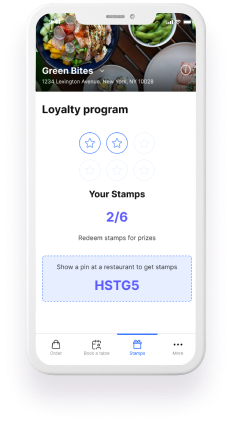The image depicts a white cell phone with visible bezels around its edges. At the top of the phone, there is a small cutout housing the front camera and a speaker, both also white. The screen displays what appears to be an advertisement or informational page, likely related to a restaurant or food product organization.

At the very top-right corner of the screen, there are indicators for battery life and cellular signal strength, accompanied by another faint and indistinguishable icon. Similarly, a few indistinct icons are found at the top-left corner. The top portion of the screen shows a border image featuring several dishes. The image includes a salad on a blue plate, various vegetables in a white bowl, and two additional white plates that are empty.

Text on the screen reads "Green Bites" in white, along with an address. Just below, there is a section detailing a loyalty program, which states "Your stamps: 2 of 6" and "Redeem stamps for prizes." Instructions to "Show pin at the restaurant to get stamps" follow, along with a code "HST G5."

At the bottom of the screen, typical cell phone navigation icons are visible.